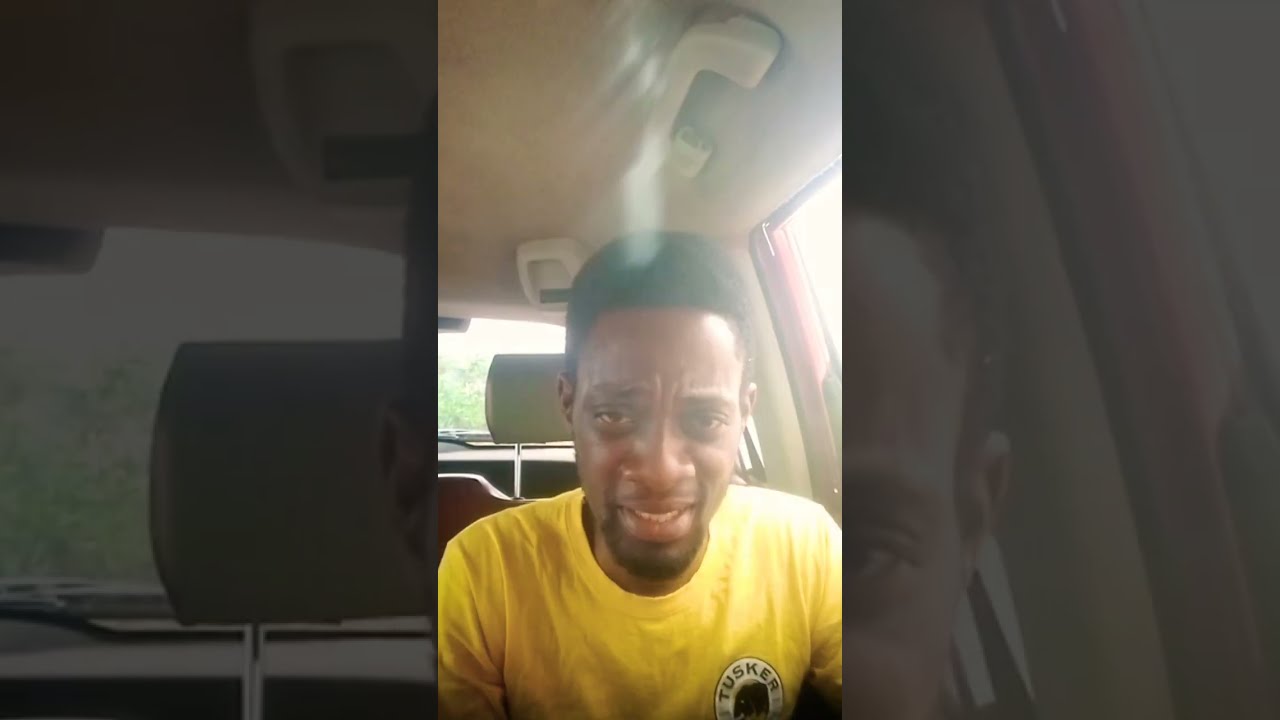In this image, an African American man is seated in the back of a car, illuminated by daylight streaming through the windows. The car’s interior features light tan upholstery. The man has a short afro and a black goatee. He is wearing a bright yellow t-shirt with a Tusker logo on the left breast, consisting of a black circle with white lettering. Positioned near the center of the photo, he gazes directly at the camera with a furrowed brow, partially closed, squinting eyes, and a slightly open mouth, conveying a look of concern or upset. The background reveals the top of the headrest from the car seat and trees visible through the rear windshield. A handle is located above him on the ceiling.